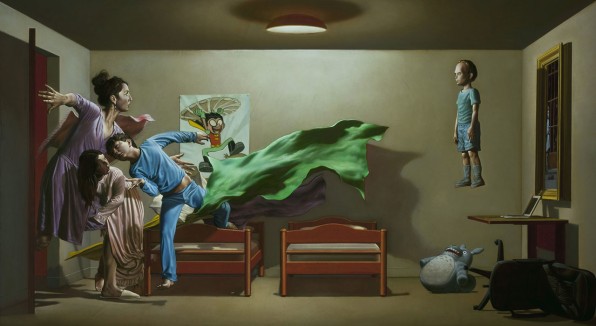In this surreal computer-generated illustration, a family scene unfolds in a shared children's bedroom with brown walls. The mother, dressed in a purple nightgown with black hair tied up in a bun, stands by an open door on the left side of the room, having just entered. Two twin-size beds with wooden frames are positioned in the middle of the room, their green and purple blankets levitating mysteriously in the air. Above the beds, a feather is floating, adding to the surreal atmosphere.

On the right side, a window with a yellow frame allows light into the room. Beneath it, an office chair lies overturned beside a small table with a laptop computer and a stuffed animal. The central focus is on a young boy in a blue-green shirt and shorts, who is astonishingly hovering in the air near the window, displaying apparent telekinetic powers. A cartoon poster resembling Robin from Batman and Robin decorates the wall behind him.

The girl's figure, dressed in a pink robe, is twisted toward the floating boy, partially facing the viewer. The boy in blue pajamas appears to be leaping out of bed, running away in surprise or excitement. The mother, her arms outstretched, watches in a mix of shock and awe as her children appear to levitate, captivated by the supernatural occurrence unfolding in their otherwise ordinary bedroom.